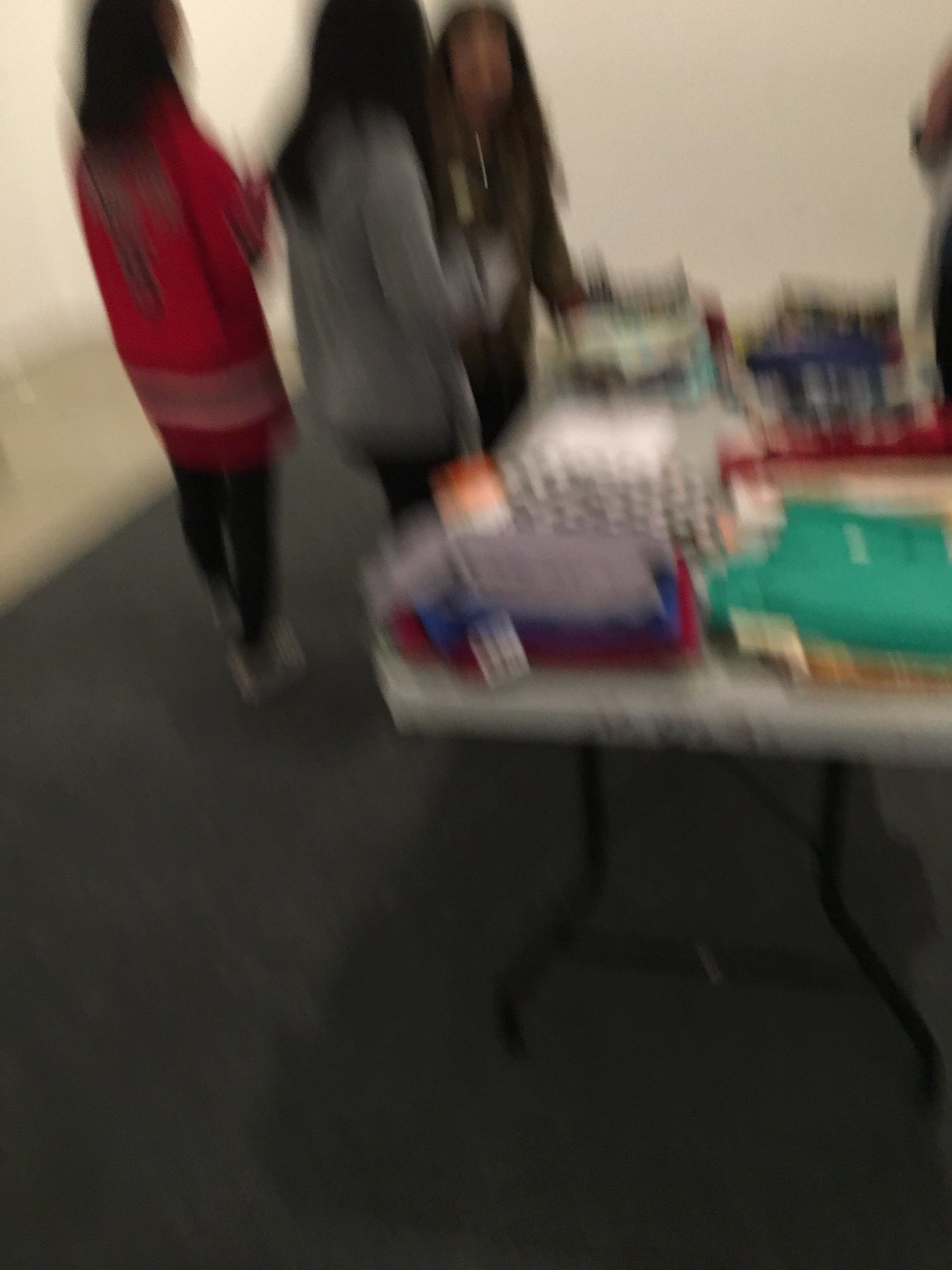The image, though very blurry, depicts a scene in a room with white walls and gray carpet. Central to the image is a metal folding table with a white tabletop and black legs, positioned towards the center-right of the photo. The table is covered in neatly folded clothing of various colors, including green, gray, blue, red, and black, with visible tags dangling from some items, suggesting a setting like a bazaar, garage sale, or clothing clearance.

Three women, all with dark hair, are present in the scene. To the left, a woman stands with her back to the camera, wearing a long red jersey with black lettering and black leggings paired with tennis shoes. Next to her, another woman also has her back turned. She has long brown hair and is dressed in a long-sleeve gray shirt and black pants. Standing in front of these two, facing the camera, is a third woman. She sports a long-sleeve brown shirt and has long brown hair, but her features are difficult to discern due to the blurriness of the image. The women's attire and positioning suggest they are either browsing or organizing the clothing on the table.